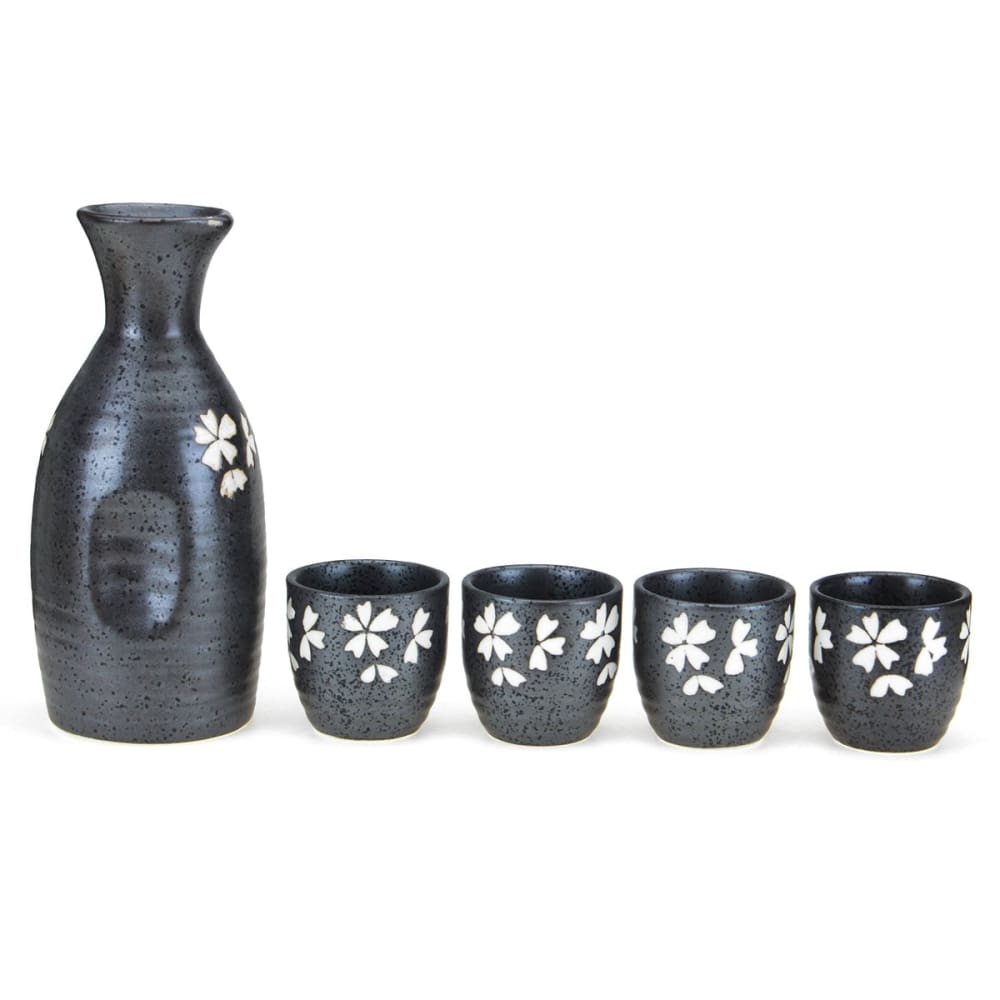The image depicts a set against a stark white background, featuring a large, vase-shaped jug positioned on the left and four smaller drinking cups to its right, all meticulously aligned in a row. The jug, reminiscent of a carafe or pitcher, has a dark gray, almost charcoal hue with numerous pockmarks and speckles covering its surface. It boasts a tapered, thinner neck adorned with a few white cherry blossom flowers towards the right side, each with distinct five-petal patterns. The jug also includes indents along its sides to facilitate easy grip.

The four accompanying cups, which are noticeably shorter and handle-less, mimic the jug's material and color scheme. These small cups, bearing a resemblance to shot glasses, are similarly dark gray with black speckles. Each cup is embellished with multiple white cherry blossom flowers near the rim, echoing the floral design found on the jug. Together, the set exudes an Asian-inspired aesthetic, unified by the consistent use of speckled gray clay and delicate floral motifs.